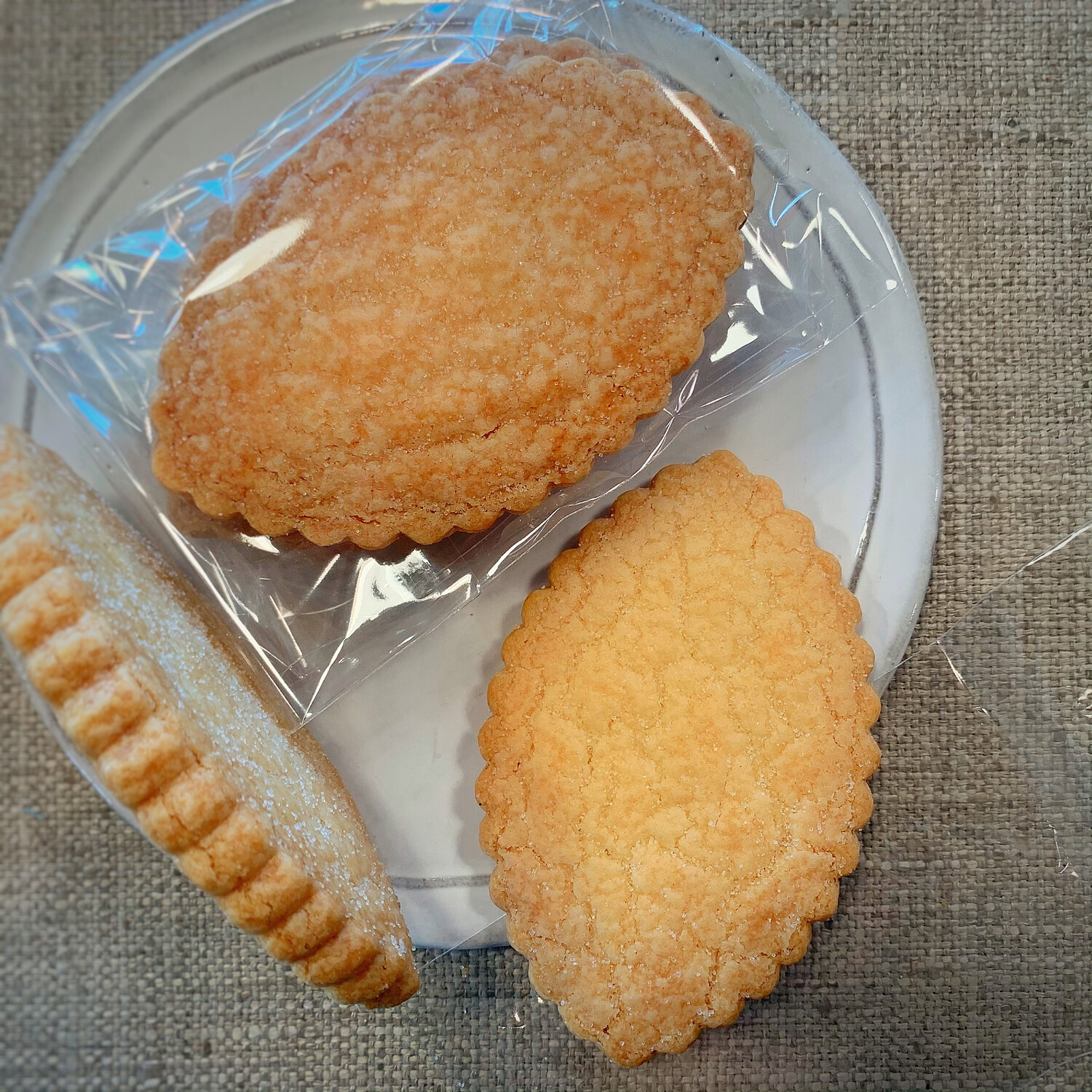The horizontal rectangular close-up image showcases a selection of cookies arranged on a circular white plate with a silver band near the edge, sitting on a textured, brown fabric that could be either a tablecloth or couch cushion. In the upper left corner of the image, there's a cookie still wrapped in a cellophane wrapper placed on the plate. Adjacent to it lies an unwrapped cookie that appears identical to the wrapped one. Below these, slightly to the lower left, is another cookie standing on its edge, featuring a scalloped border and a dusting of powdered sugar—unlike the flat-lying cookies, which lack powdered sugar. The cookies form a triangular arrangement, with colors in the image comprising various shades of brown, gray, yellow, orange, white, and touches of black. The overall impression suggests a casual, homey setting.